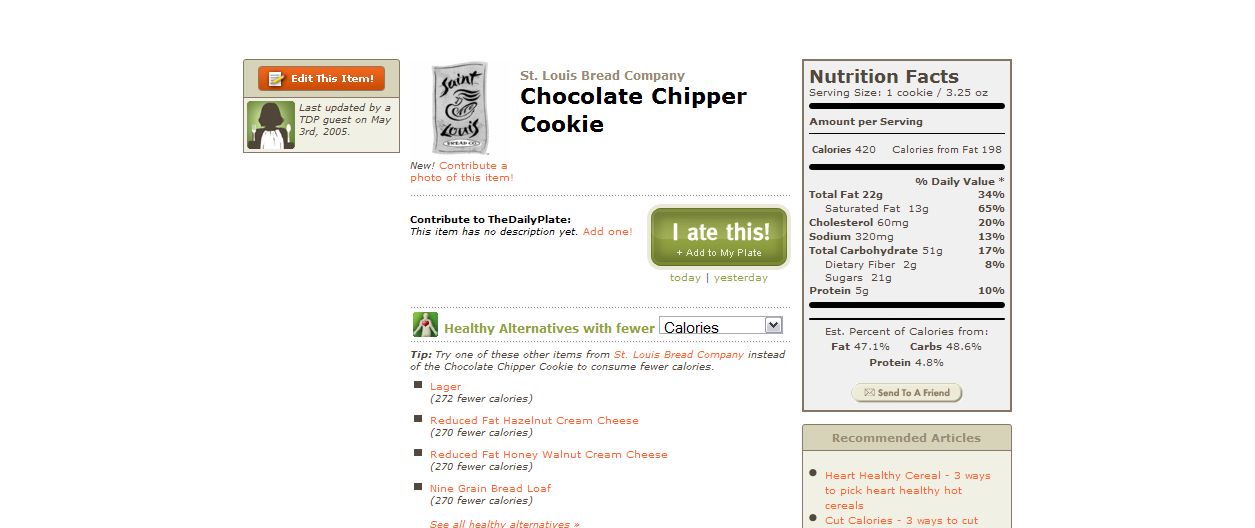The series of three images depicts an old-school early 2000s-style website focused on nutritional information and healthier alternatives for various food items. The first image displays an editable page last updated by a guest in May 2005, featuring a St. Louis Bread Company chocolate chip cookie. The second image shows the cookie in question and includes a feature for users to upload photos, add reviews, or comment. There's a green button labeled "I ate this," emphasizing user engagement. The website suggests healthier alternatives with fewer calories, and other detailed metrics can also be selected. The final image contains the nutrition facts for the cookie, which weighs 3.25 ounces and contains 420 calories, 198 of which are from fat. The nutrition facts are detailed, listing total fat as 22 grams (34% DV), saturated fat at 13 grams (65% DV), cholesterol at 60 milligrams (20% DV), sodium at 320 milligrams (13% DV), total carbohydrates at 51 grams (17% DV), dietary fiber at 2 grams (8% DV), sugars at 21 grams, and protein at 5 grams (10% DV). Below these facts, the website offers recommended articles and similar items such as reduced-fat variations. The nostalgic layout and comprehensive features suggest it's a resource for users seeking detailed nutritional info and healthier eating options.